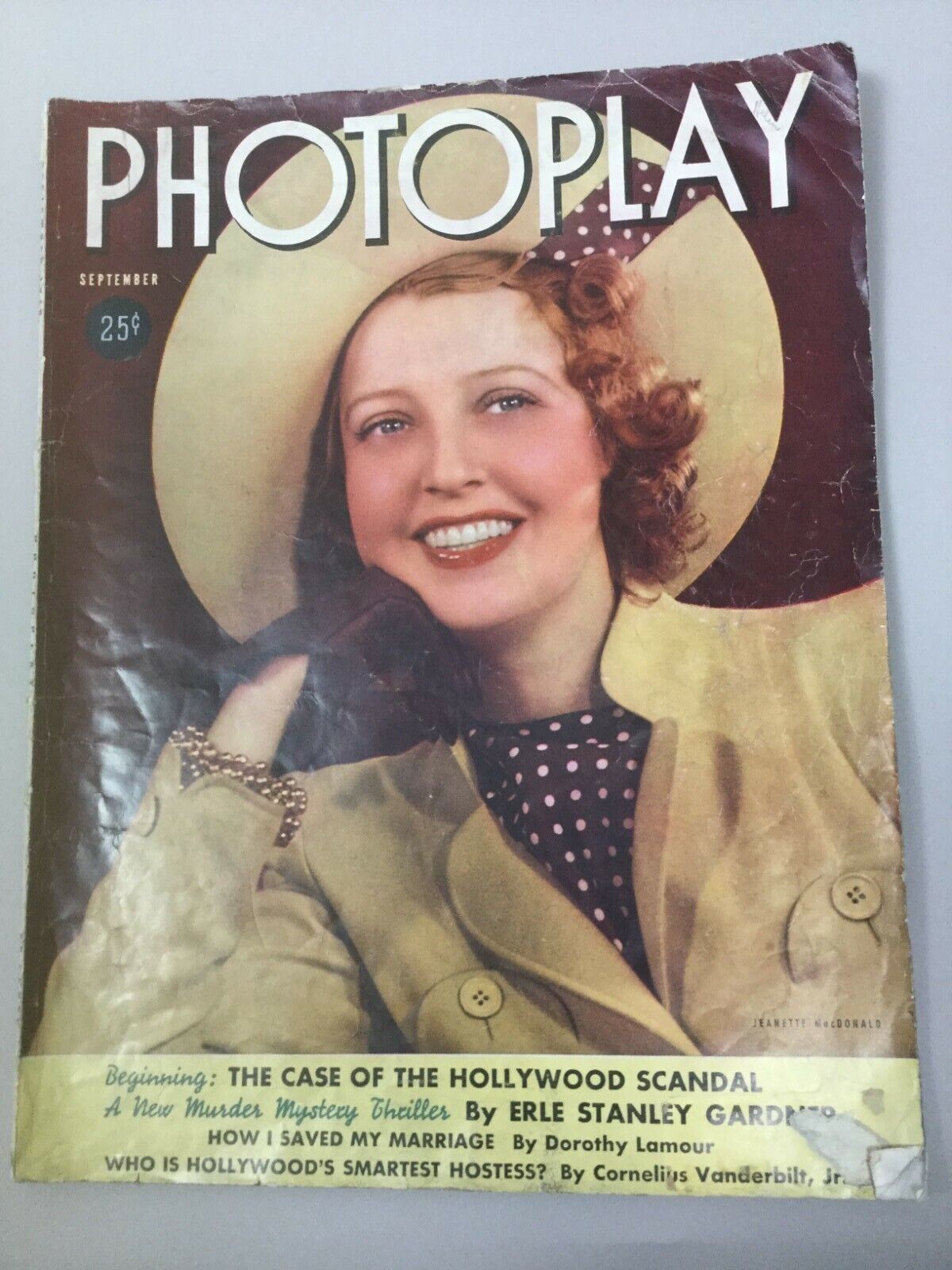This vintage magazine cover titled "Photo Play" appears to be from September, priced at 25 cents. The layout is in a portrait orientation with a gray background outside the cover. The main background color of the cover itself is brown. The central focus of the image is a woman showcased from the chest up. She has red curly hair cascading to her chin and is adorned with a small cream hat adorned with a brown ribbon featuring white polka dots. Her right hand, clad in a black or brown leather glove, rests elegantly against her face as she smiles warmly, revealing white teeth and red lipstick, while her blue eyes gaze forward.

She wears a brown shirt spotted with white polka dots, under a cream jacket, and sports a notable gold bracelet around her wrist. At the very bottom of the cover, there's a yellow bar with black text. Notable headlines on the cover include a feature by Earl Stanley Gardner titled "The Case of the Hollywood Scandal," "How I Saved My Marriage" by Dorothy Lamore, and "Who is Hollywood’s Smartest Hostess?" by Cornelius Vanderbilt Jr. The text at the bottom is primarily in black, set on a yellowish background. The vintage styling evokes a sense of an old Hollywood era, reminiscent of the more conservative and tasteful fashion trends of the past.